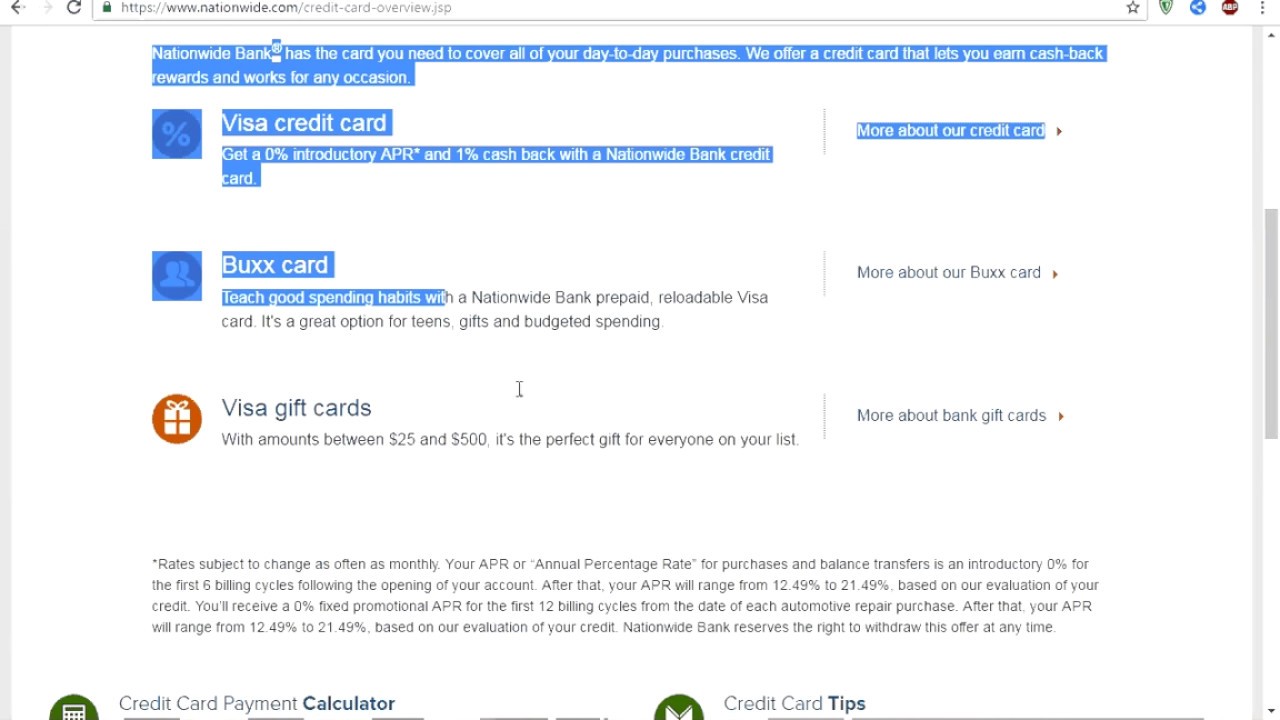The image displays a webpage focused on Visa gift cards. A prominent Visa credit card is shown alongside a section of box-style cards, both highlighted in blue. The webpage is open in an unidentified browser, and a hyperlink labeled "Visa Gift Cards" is clearly visible. There is some additional text on the page. On the left side, a gray scrollbar indicates that the viewer is approximately halfway down the page. The gray bar is about 200 pixels in height.